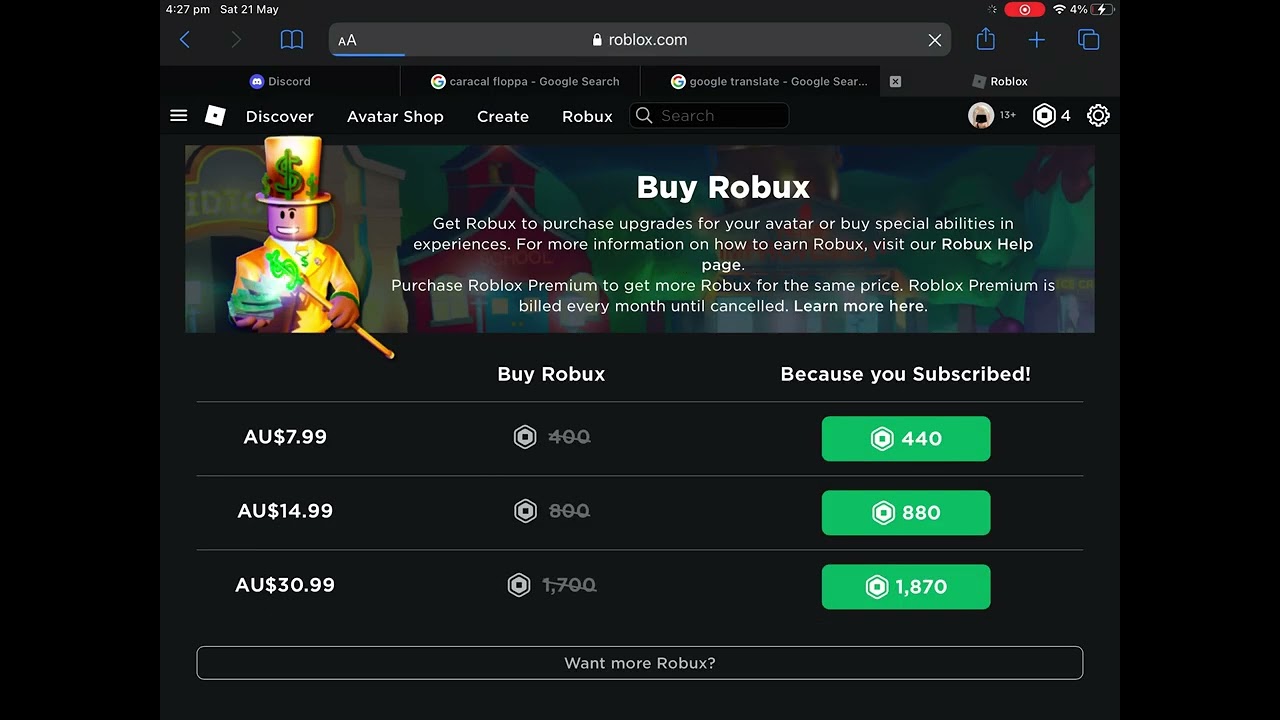Screenshot of a Roblox Web Page on a Mobile Device

The image is a screenshot from the game Roblox, viewed on a mobile device or potentially an iPad. The interface elements indicate the device is charging, with the battery at 4% and a little lightning bolt symbol. The status bar also displays the time as 4:27 PM on Saturday, May 21st, and shows a strong Wi-Fi connection. There is a red stop button indicating screen recording is in progress.

The webpage is displayed in dark mode, featuring a black background with white text. At the top, the URL bar shows "roblox.com" with a padlock icon, signifying a secure connection. On the left side of the address bar, there are small and large 'A' icons for adjusting the reader view, which facilitates text-only browsing. To the right of the URL box, there is an 'X' button to stop the current activity. Additional navigation icons include blue arrows for back and forward navigation, a bookmark icon that resembles a book, a share icon depicted as a square with an arrow pointing up, a plus sign for opening new tabs, and a copy icon represented by two overlapping pieces of paper.

Beneath the navigation bar, the main content of the Roblox page includes a prominent banner advertising "Buy Robux." The banner explains that Robux can be used to purchase upgrades for your avatar or special abilities in experiences. Detailed information about earning Robux can be found on the Robux help page. The ad also mentions Roblox Premium, which provides more Robux for the same price and is billed monthly until canceled.

An image of a Roblox avatar wearing a gold top hat and jacket accompanies the text. Pricing details in Australian dollars are provided: $7.99 for 440 Robux, $14.99 for 880 Robux, and a special offer of $13.99 for 1,870 Robux for subscribers. The final line of the advertisement invites users to "Want More Robux."

This detailed screenshot effectively captures the various elements displayed on the Roblox webpage, emphasizing the dark mode interface, the promotional banner, and the different navigation and functional icons within the mobile browser.